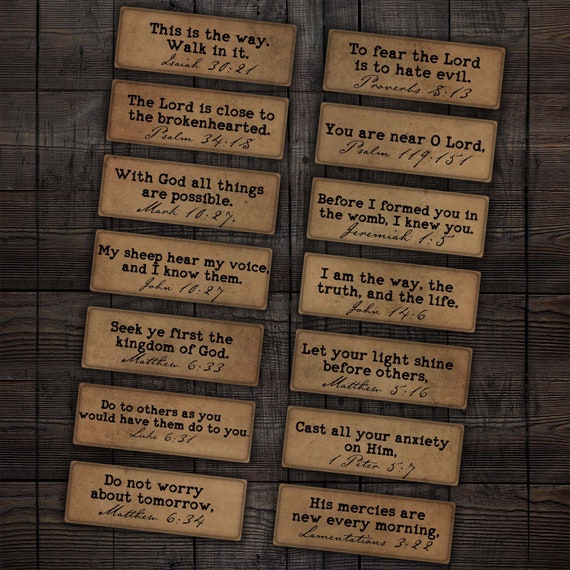The image depicts a dark wooden background, possibly a table or wall, with two columns of small wooden plaques aligned vertically and slightly angled to the right. Each plaque bears a religious message or Bible verse printed in black lettering. On the left column, from top to bottom, the plaques read: "This is the way. Walk in it," "The Lord is close to the brokenhearted," "With God, all things are possible," "My sheep hear my voice and I know them," "Seek ye first the kingdom of God," "Do to others as you would have them do to you," and "Do not worry about tomorrow." On the right column, from top to bottom, the plaques read: "To fear the Lord is to hate evil," "You are near, O Lord," "Before I formed you in the womb, I knew you," "I am the way, the truth, and the life," "Let your light shine before others," "Cast all your anxiety on him," and "His mercies are new every morning."